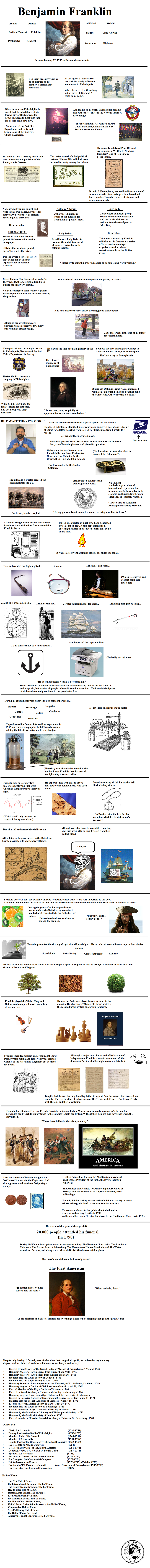This image appears to be a blurred timeline of Benjamin Franklin's life, with the only legible text being his name. The image is difficult to interpret due to its poor quality, making the pictures and detailed writing indistinguishable. Among the discernible elements is an anchor, which could be related to Franklin's inventions or significant events in his life. The timeline features a variety of colors, but their specific significance remains unclear. The overall presentation is perplexing, as the quality diminishes the intended informative value of the display.